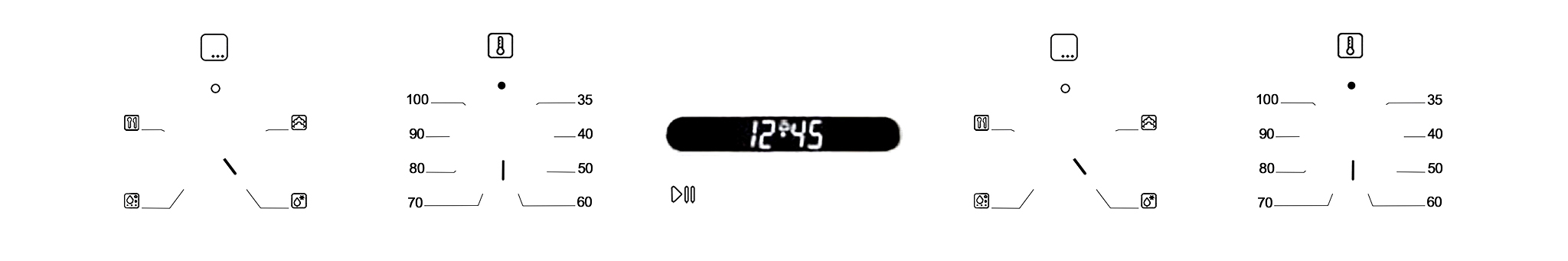This image appears to be a template for printouts, possibly for use on a thermostat or similar electronic device. 

The template consists of three main sections:

1. **Leftmost Section**: This area displays five squares arranged in a star-like pattern, each connected by lines. Various icons are also present, though their specific details are not mentioned.

2. **Middle Section**: Dominated by a black bar, this section shows the numbers "12" and "45," possibly indicating time or a different measurement, alongside a set of media control icons: play, pause, and two additional icons identical on either side of the central pair.

3. **Rightmost Section**: This section has a small temperature icon at the top. Along the left side, it lists the numbers "190, 80, 70," and along the right side, it displays "35, 40, 50, 60," each connected by lines, likely indicating temperature ranges or settings.

Overall, the template combines visual elements for potentially controlling and displaying information related to a thermostat or a similar device.